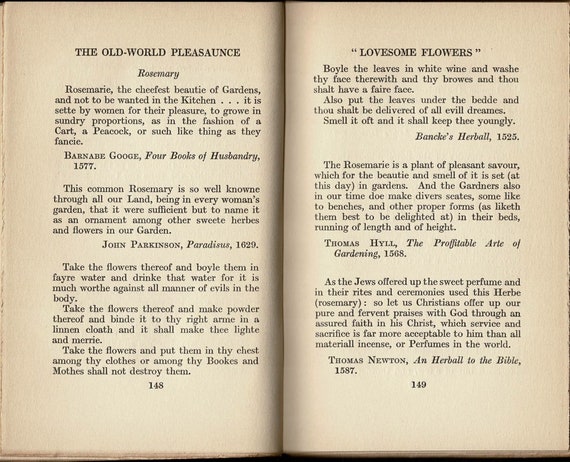The image features an open book, displaying pages 148 and 149. The book's title, "The Old World Pleasaunce," is written on the top left of page 148. The chapter title, "Lovesome Flowers," is on the top right of page 149. Each page exhibits an array of short paragraphs filled with quotes about rosemary from various historical texts. 

On page 148, the first paragraph highlights rosemary as "the chiefest beauty of gardens, and not to be wanted in the kitchen," with an attribution to Barnard Gouge's "Four Books of Husbandry," published in 1577. The subsequent paragraphs include quotes from John Parkinson's "Paradise" (1629), extolling rosemary's virtues for health and household uses, such as boiling and drinking its flowers for medicinal purposes. The page concludes with practical advice for using rosemary as both a moth repellent and a cheerful herb.

Page 149 continues with the benefits and applications of rosemary. It mentions medicinal uses such as boiling leaves in white wine to wash the face for a fair complexion and placing leaves under the bed to ward off bad dreams. Quotes from "Banky's Herbal" (1525), Thomas Heibel’s "The Profitable Art of Gardening" (1568), and Thomas Newton’s "An Herbal to the Bible" (1587) further elaborate on rosemary's historical significance, fragrance, and symbolisms in garden aesthetics and religious rites. Each paragraph emphasizes the enduring charm and utility of rosemary through centuries-old perspectives.

The detailed references to years and diverse historical texts underscore the enduring admiration and multifaceted uses of rosemary, blending horticultural beauty with practical and ceremonial applications.